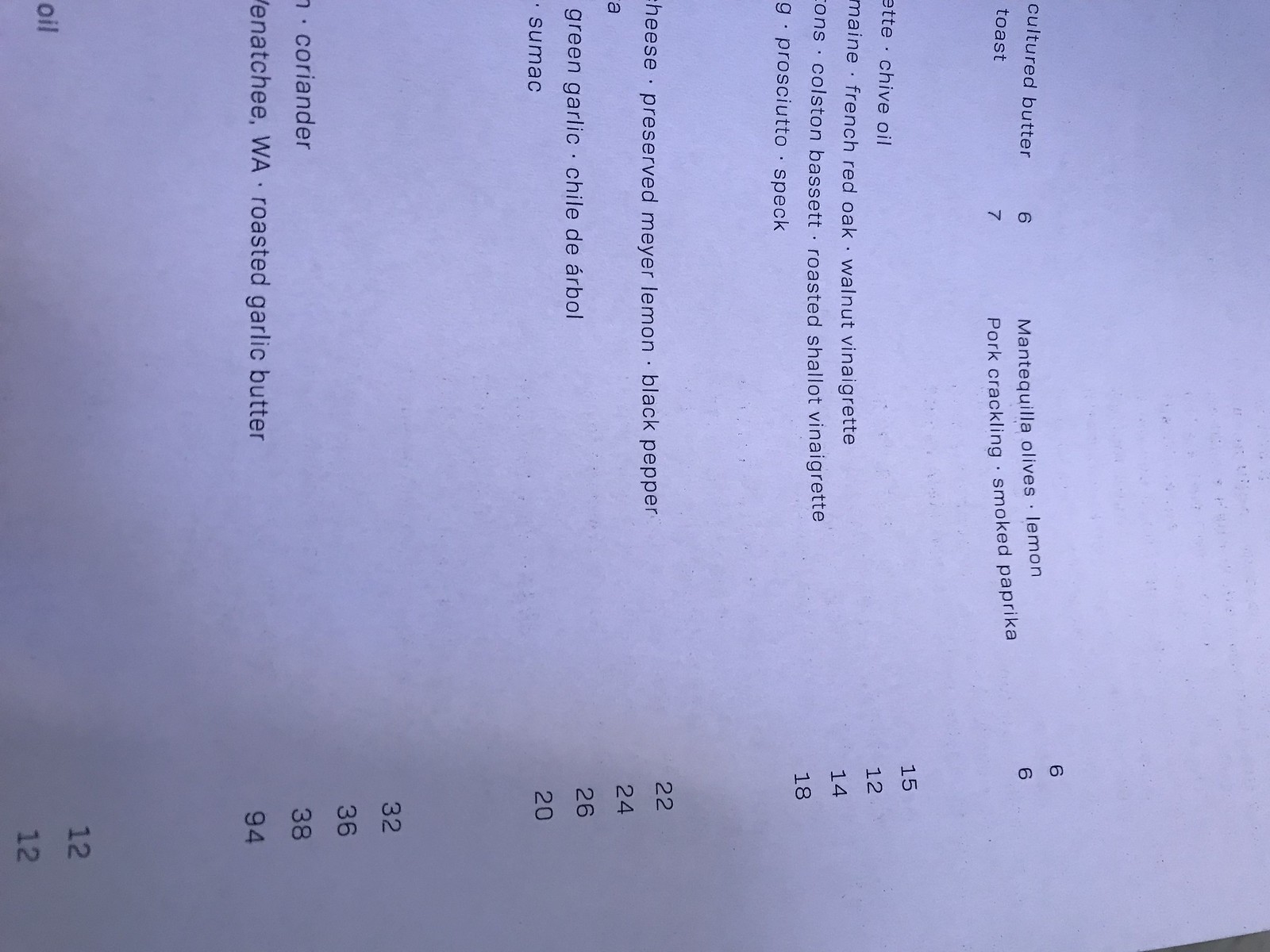The image features a close-up photograph of a sheet of paper containing black text, which is positioned horizontally in the frame, causing the text to appear sideways. The sheet of paper dominates the image, with a small portion in the bottom right corner showing an indistinct gray area beyond the edge of the paper. The text on the paper includes a list of food items along with their corresponding prices. The visible text at the top of the page reads "mantequilla olives," "lemon," "pork crackling," and "smoked paprika," indicating that this is a menu. The prices are listed in a vertical sequence on the right side of the paper, reading as follows: 6, 6, 15, 12, 14, 18, 22, 24, 26, 20, 32, 36, 38, 94, 12, and 12.